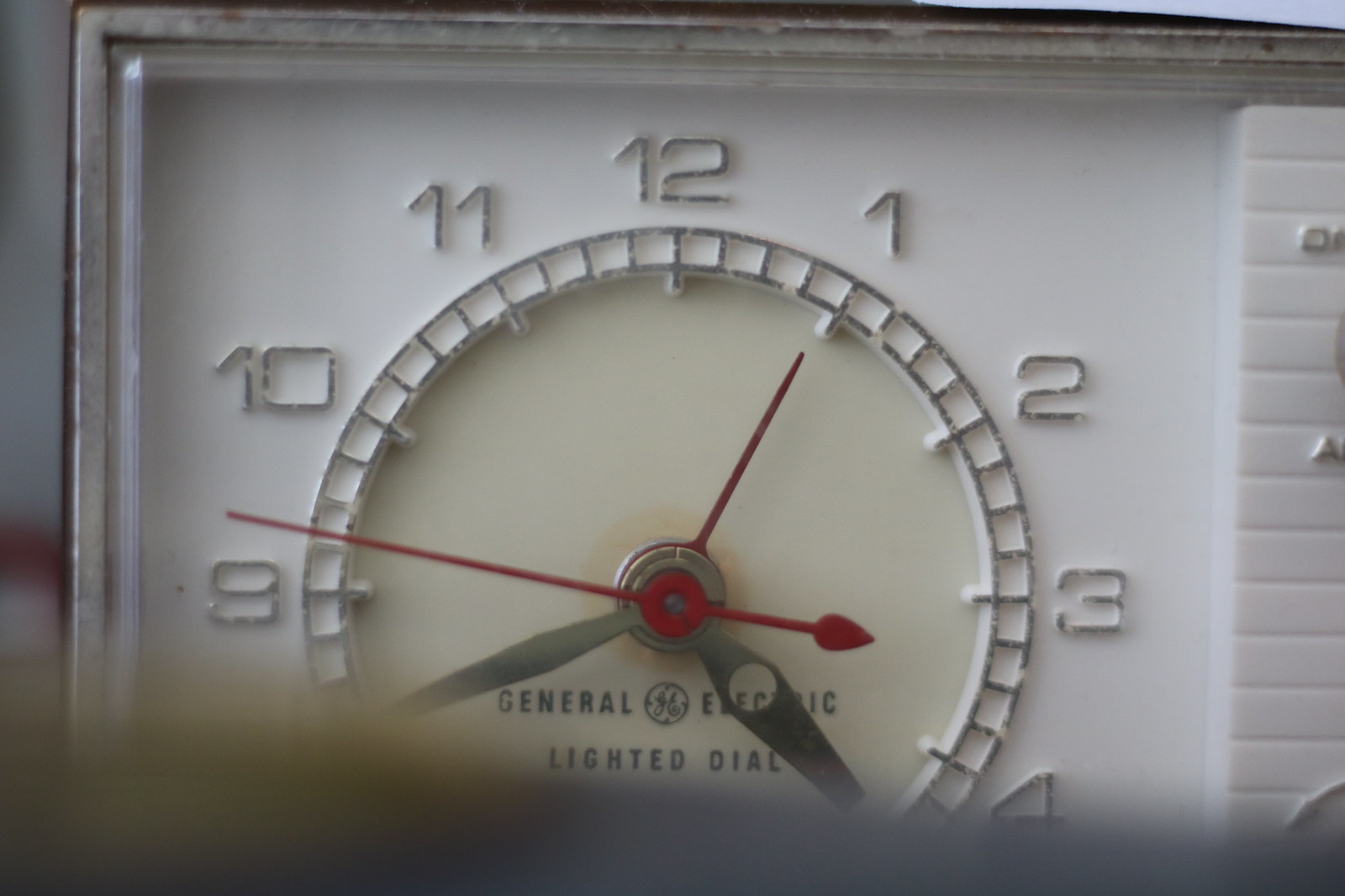This photograph showcases a vintage General Electric clock, notable for its illuminated dial. The clock features a logo indicating its GE brand, with stylistic elements suggesting it dates back to the 1980s or earlier. The numerals are embossed on white plastic and painted in silver, though time has caused wear and fading across the clock face. The hour and minute hands are crafted from silver, while the red second hand appears to be made of plastic. Encircling the clock face is a white plastic frame, further bordered by a metallic rim, adding to the antique charm of the piece.